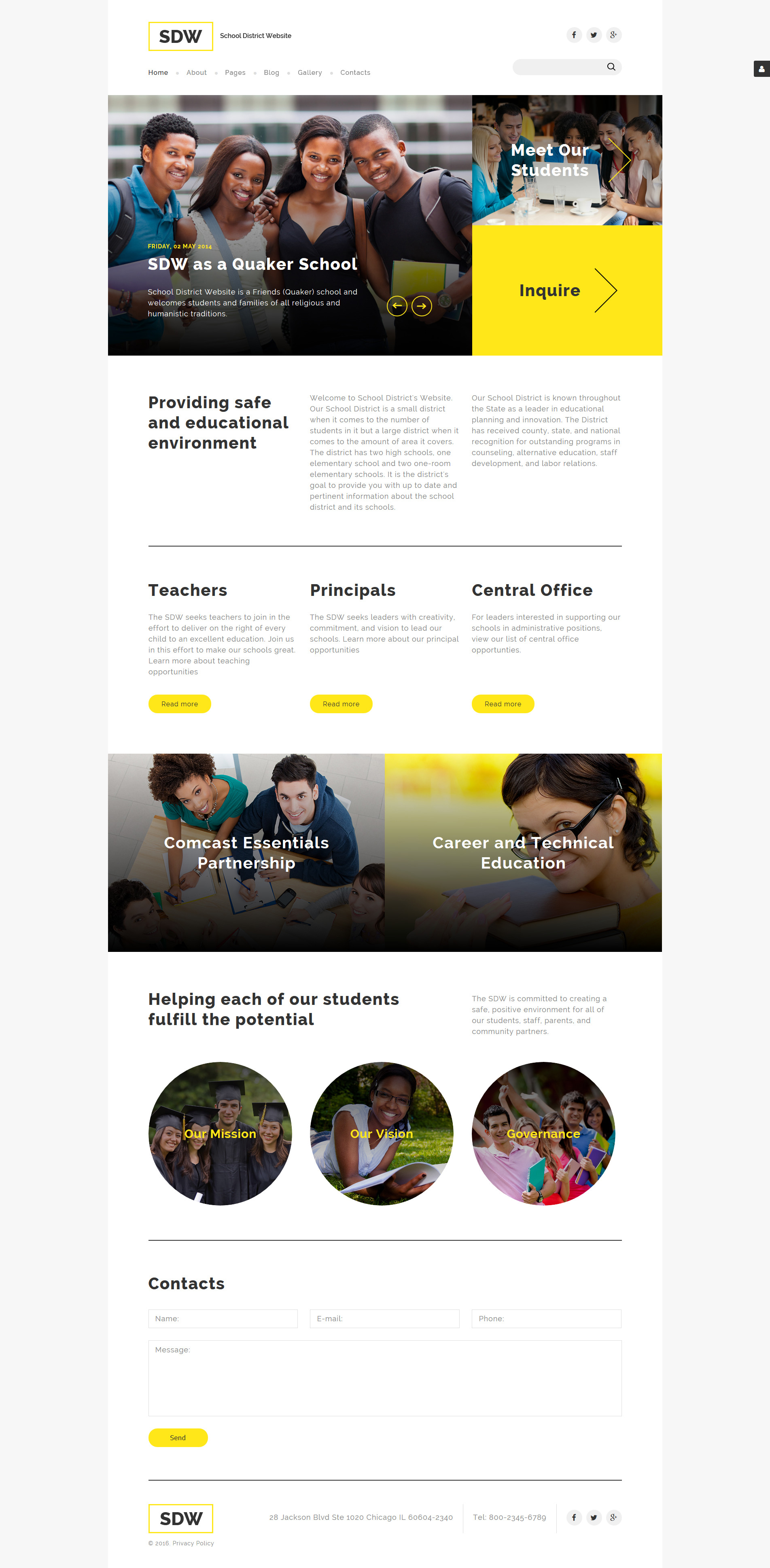This screenshot appears to be an advertisement embedded within a web page, likely from an educational institution. The central area of the screenshot displays the webpage bordered by grey bars on either side. The webpage itself has a clean design with a white background.

At the top, there's a prominent yellow rectangle featuring the text "SDW" in black font. Adjacent to this, there's additional black text that is indiscernible due to its small size. Beside the text are icons for sharing the content on Facebook, Twitter, and Pinterest.

Below this header area, there's a navigation menu with several clickable options, though the text is too small to decipher. 

The main section of the webpage features a photo of four smiling black college students, standing and looking at the camera. On the left, a male student with a backpack poses next to two female students wearing dresses. On the far right, another male student with a backpack completes the group.

To the right of the photo is a button labeled "Meet Our Students," which is clickable. Directly below this is another clickable yellow button labeled "Inquire."

Further down, there's a paragraph with the heading "Providing a Safe and Educational Environment," written in black font on a white background. However, the detailed content of the paragraph is too small to be legible.

At the bottom of the screenshot, there are clickable links labeled "Teachers," "Principals," and "Central Office," likely leading to more detailed sections of the website.